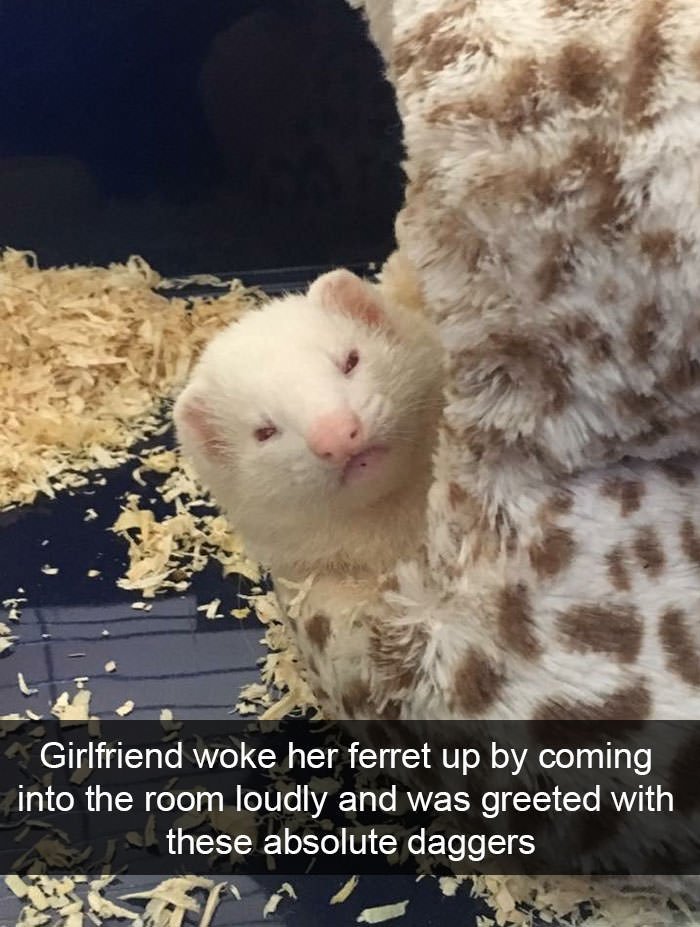The photograph captures a white ferret with a pink nose and ears, glaring angrily at the camera with narrowed eyes. The ferret's head is poking out from a plush quilt or bed that features a leopard print pattern with brown spots on white, hairy fabric. Set against a navy blue and black background, the ferret’s reflection is visible on the shiny base of its clear container. Scattered pine or wood shavings, light in color, are seen in the background, contributing to the ferret cage setting. At the bottom of the image, a semi-transparent black banner with white text reads, "Girlfriend woke her ferret up by coming into the room loudly and was greeted with these absolute daggers." This detailed portrait captures a moment of the ferret’s apparent irritation, blending realism with textual elements.